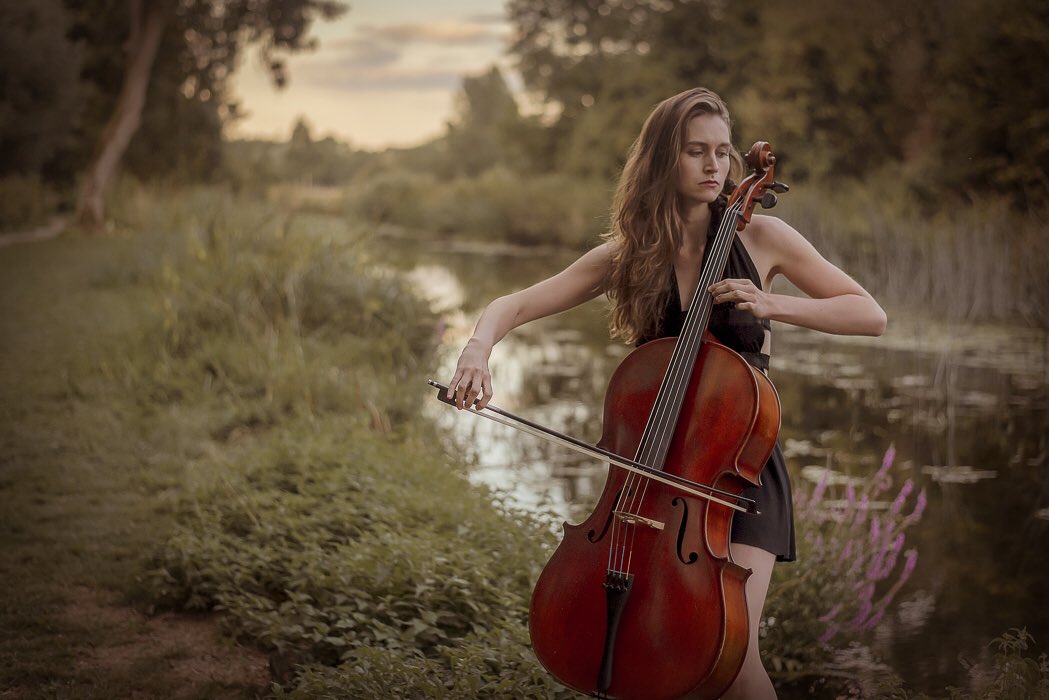The photograph depicts a young woman, approximately 18 years old, elegantly playing a cello in an outdoor setting by the banks of a narrow, winding creek. Her long, wavy brown hair cascades down her back, almost reaching her waist. She wears a black sleeveless mini dress that accentuates her statuesque posture as she stands facing the camera, her head subtly turned to the right. Her right hand wields the bow, striking the cello strings, while her left hand is positioned on the fingerboard, delicately plucking and forming chords.

The tranquil background adds depth and serenity to the scene. Tall grasses with occasional pink blossoms line the creek banks, interspersed with low-lying shrubs and the looming presence of dark green trees. The water in the creek is remarkably still, adorned with lily pads and patches of algae. Above, a gray sky with patches of brightness peeks through the foliage, hinting at an overcast day. The overall composition blends natural elements and artistic performance in a harmonious tableau.